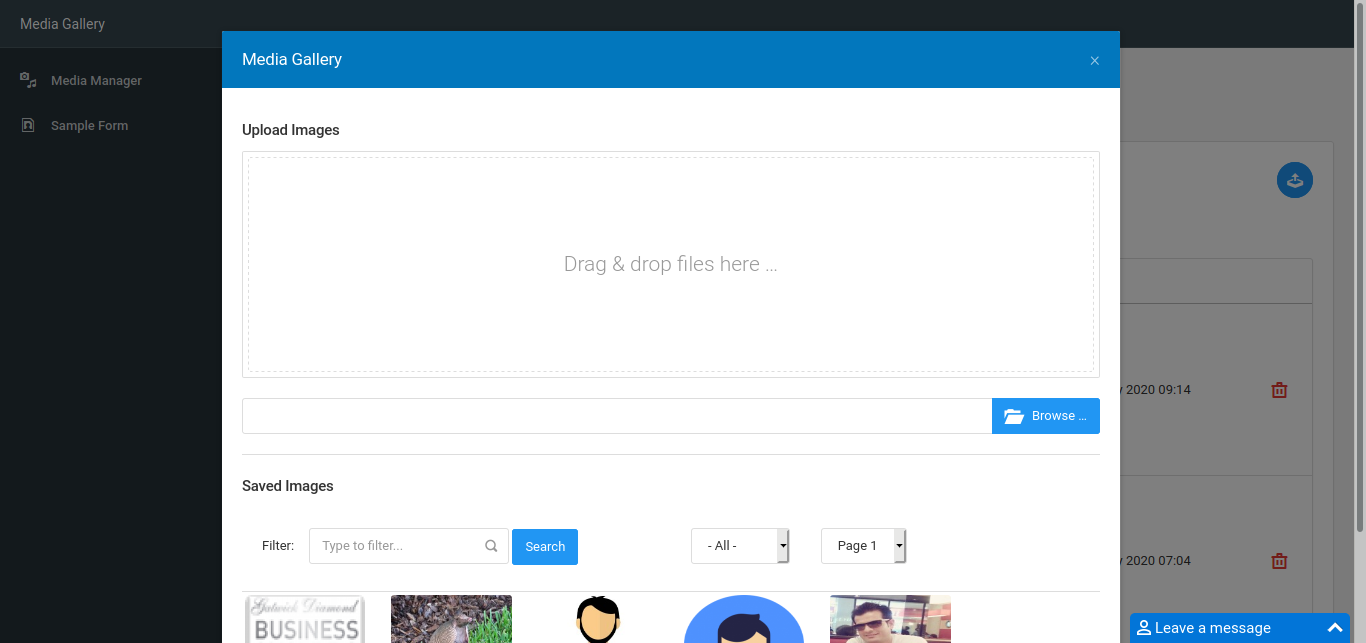The image depicts a computer monitor displaying a media gallery interface. In the foreground, a large rectangular pop-up window occupies the majority of the screen, prompting the user to "Upload Images." Within this box, there are instructions to "Drag and Drop Files Here." Below this main area is a gray box with a blue folder icon on the right-hand side, labeled "Browse," allowing for file selection from the computer.

Below this upload section, the interface lists "Saved Images" with options for filtering and searching through a search bar enclosed in a blue box labeled "Search." Adjacent to these filters, there are additional control buttons in rectangular boxes, including "All" and "Page 1."

At the bottom of the screen, a row of image thumbnails is partially visible, showing various pictures including one of a person wearing sunglasses and two cartoon images, though these thumbnails are cut off and only partially viewable.